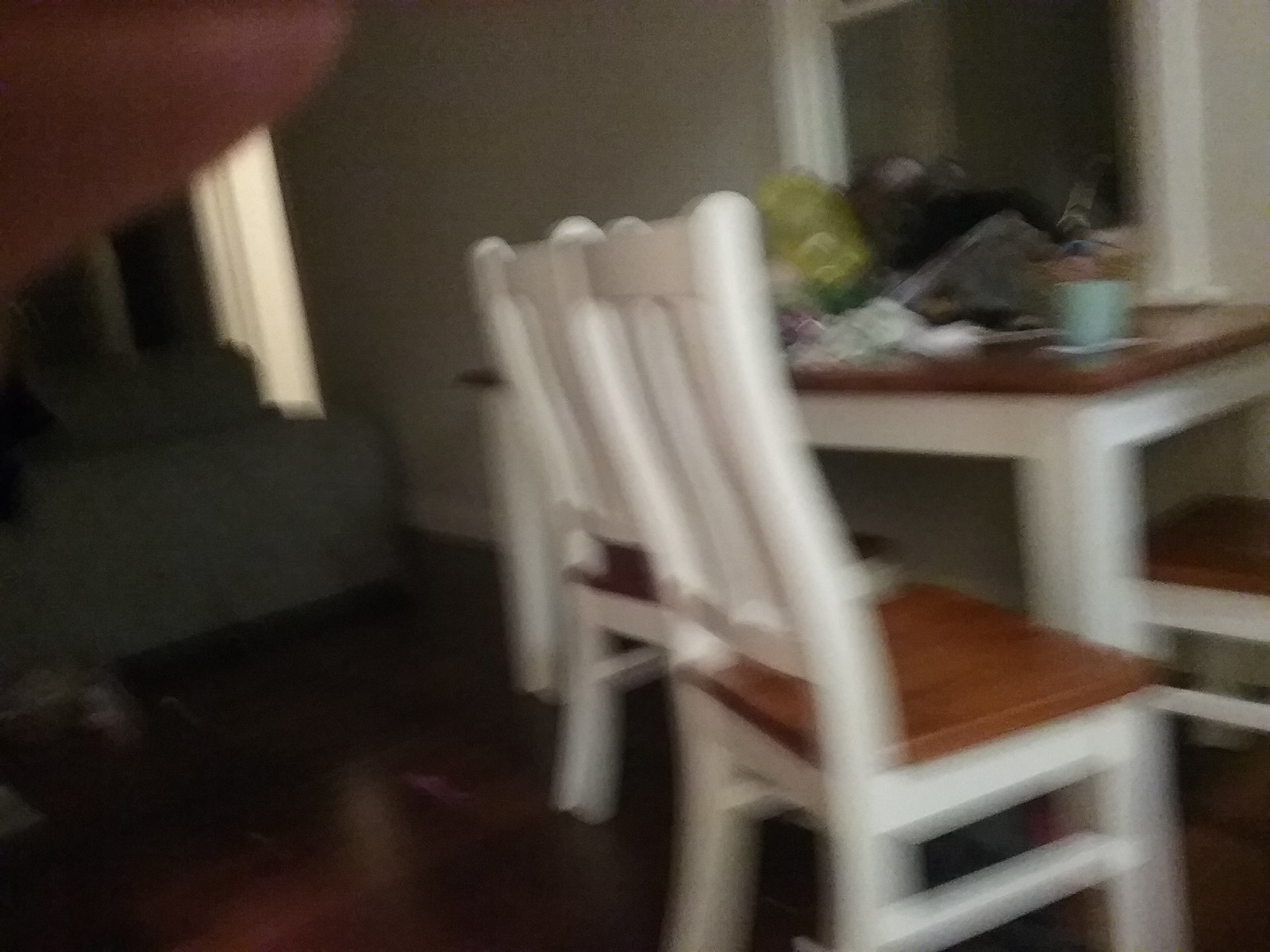A partially obscured, blurry photograph taken indoors reveals a dining or kitchenette area. The image is marred by a finger covering the upper left part of the lens. The focal point is a set of three to four chairs, one of which might be a stool partially hidden from view. The chairs feature white backs with two small slots at the center and have square, brown mahogany seats that widen at the front and narrow toward the back. The matching table has white legs and a wooden brown top, complementing the brown wooden floor. A green couch is faintly visible on the left side, amidst a cluttered scene with various items scattered across the table and floor.